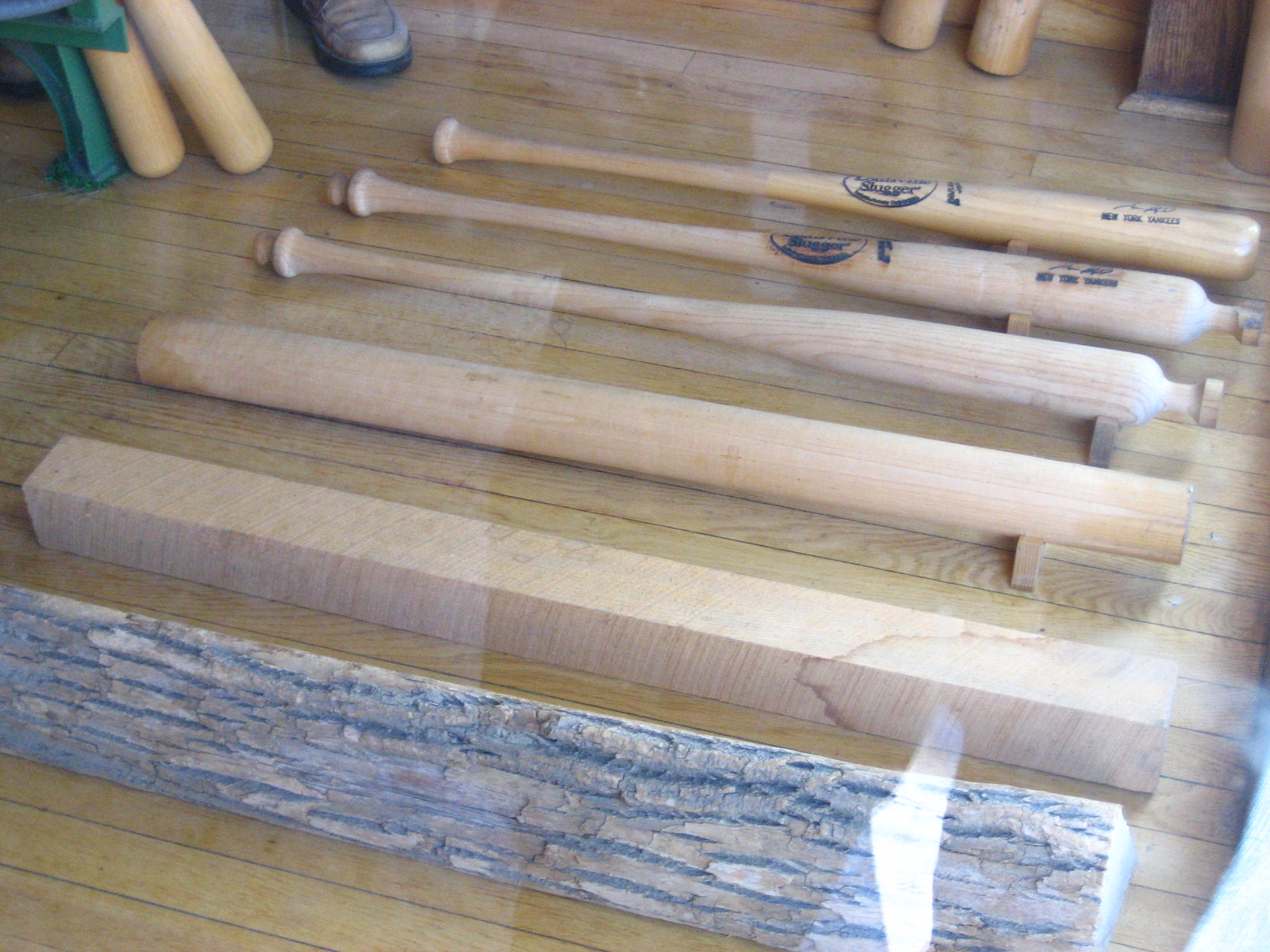This is a detailed photo showing the step-by-step process of manufacturing a baseball bat, aligned horizontally on a wooden floor. The image features six distinct stages, all facing parallel to the right. Starting from the bottom, the first object is a raw log with its bark intact. Above that, the log is cut into a smooth, square bar. The progression continues with the bar shaped into a cylinder. The next stage reveals a partially shaped bat, with lathe marks still visible. Moving further up, the bat takes on a more refined form with a handle, featuring the logo burned onto it. Finally, at the top, the completed baseball bat is displayed, varnished and polished. The background includes organized, standing baseball bats and miscellaneous items, such as a white and black shoe and something green in the top left corner.